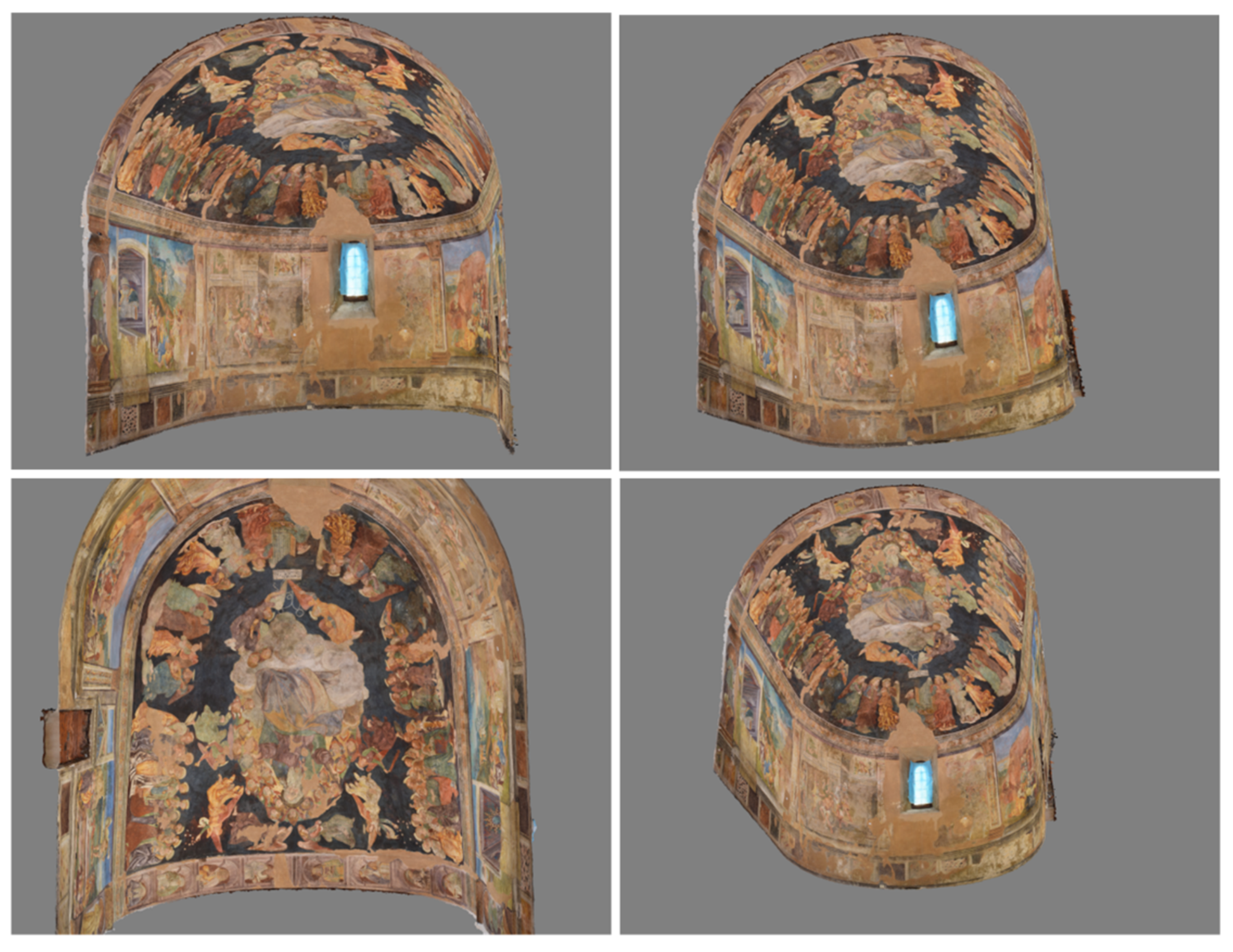The image is a four-square grid, each depicting different angles of the same 3D-rendered interior of a historic-looking cathedral or church. Dominated by warm orange and brown hues, the scene features a domed ceiling adorned with intricate Renaissance-style paintings. A window with a blue border, positioned towards the back, adds a glimmer of light to the otherwise dark interior. The perspective in each picture varies: the top left image shows the curved wall and rounded ceiling with visible brightness near the window, while the top right leans slightly to the left, offering a similar view. The bottom left photo, tilted upwards, provides a closer look at the ceiling’s ornate designs, with details of orange, yellow, and black patterns. The final image, bottom right, mirrors the second, aligning closely with the first image’s viewpoint. The cohesive color palette and repeated design elements unify the four distinct yet complementary angles, presenting a detailed and immersive view of this architectural marvel.